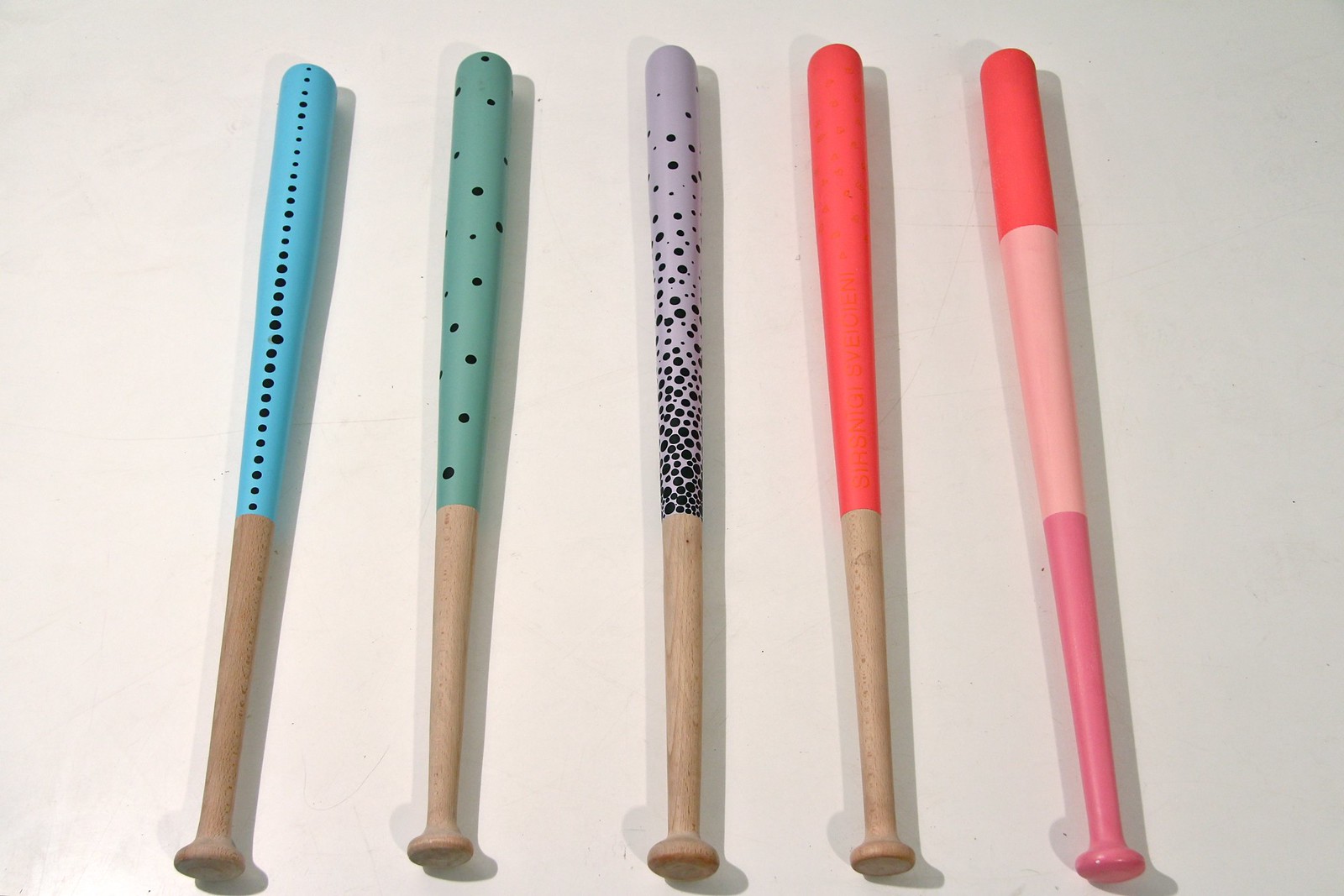This is an image showcasing five distinct, artistically painted wooden baseball bats, meticulously arranged on a white surface, with their shadows subtly cast. From left to right, the first bat is one-third natural wood from the handle and then transitions into a vibrant blue adorned with black dots. The second bat mirrors the wooden handle length but features a green upper part with randomly scattered black dots. The central bat stands out with a lavender hue, densely packed with black dots at the base, which gradually become sparser up its length. The fourth bat is a striking fluorescent coral color, completely painted with no additional designs. Finally, the bat on the far right showcases a gradient of colors with a pink handle, a lighter pink middle, and a fluorescent coral tip.